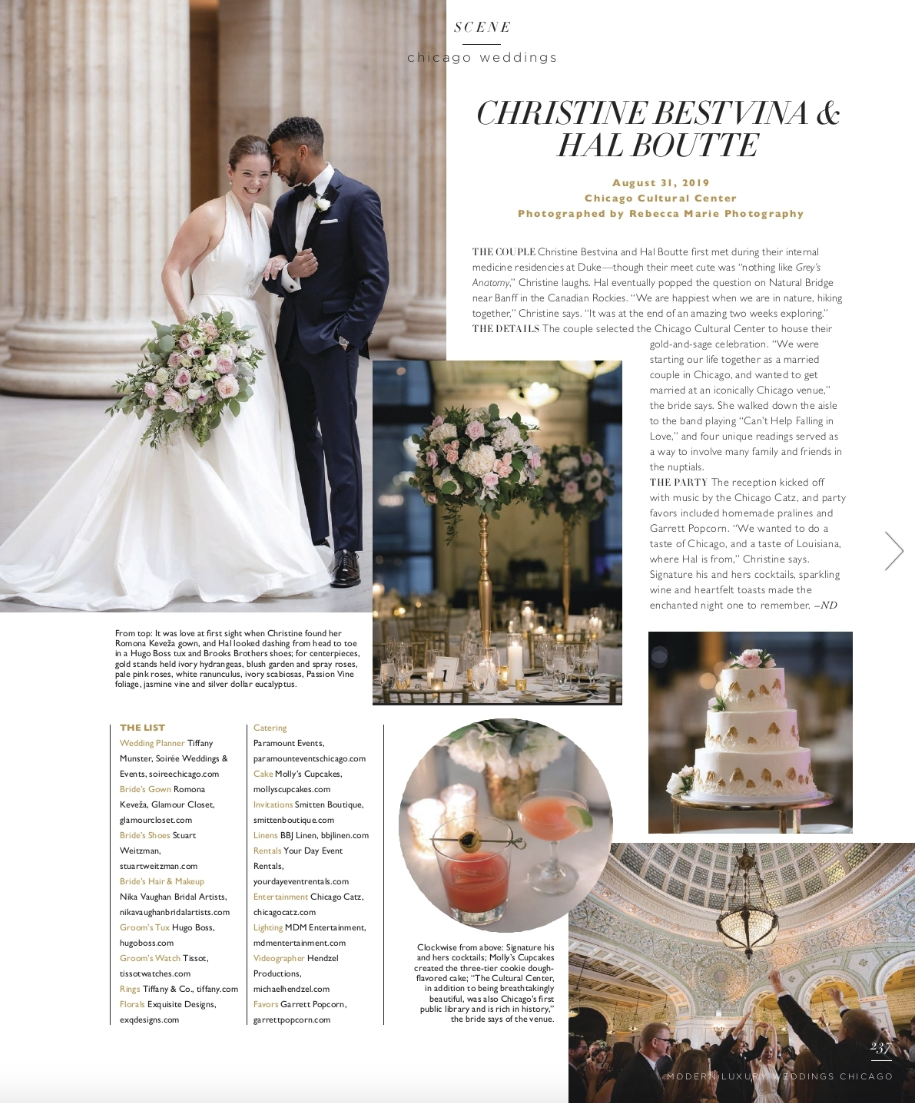The magazine page features a wedding spread headlined "Chicago Weddings," focusing on the nuptials of Christine Bestemda and Hal Boot, who tied the knot on August 31st, 2019. 

Dominating the top left corner, there's a heartwarming image of the bride and groom. The groom, dressed in a classic black tuxedo with matching shoes, gazes lovingly at his bride. She wears a simple, elegant, halter-style long white wedding gown and carries a bouquet of light pink and white flowers. The couple stands against the backdrop of a grand building with large pillars, adding an air of grandeur to the scene.

The middle section of the page includes a snapshot of the table decor, featuring golden chairs reminiscent of bamboo, tall gold bars topped with bowls of flowers, and candles enhancing the romantic ambiance. This is complemented by a circular inset showcasing the couple's specialty drinks.

To the right of these images, a three-tiered wedding cake stands proudly, symbolizing the couple's sweet union. Below, guests are captured dancing joyfully in a large hall adorned with chandeliers, celebrating the couple's happiness.

Additionally, the page includes detailed text about Christine and Hal, outlining where they met, the nature of their celebration, and acknowledging the many contributors to their special day, from the wedding planner to other key participants.